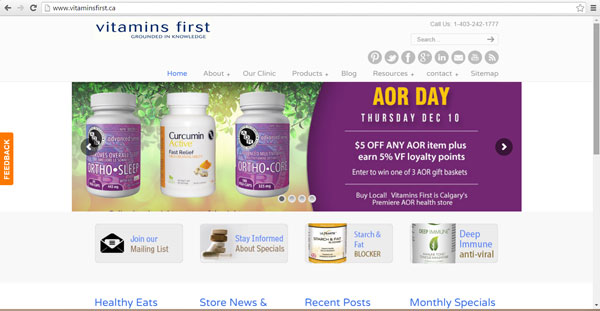A screenshot from a desktop or laptop showcases the homepage of VitaminsFirst.ca. The image is rectangular with a white background, focusing on the browser interface and website design. At the top, a thin, light gray search bar features various icons. From left to right, there is a black back arrow, a refresh icon, and within the search bar, the website URL (www.vitaminsfirst.ca) appears. To the right, there is a gray star icon and a three-line "hamburger" menu icon enclosed in a gray square.

Below the browser elements, the website’s name "vitamin first" is displayed in dark blue, lowercase letters, followed by the tagline "grounded in knowledge" in small text. On the right, in light gray, there is a contact number: "Call us: 143-242-1777". 

A secondary gray rectangular search bar with light gray text "search" and a gray arrow on its right is below the website name. Adjacent are eight circular social media icons, representing platforms like Pinterest, Twitter, Facebook, Google+, LinkedIn, and three indistinct ones.

Below this section, the navigation bar features links in a mix of blue and gray text: "home" (blue), "about", "our clinic", "products", "blog", "resources", "contact", "sitemap" (all gray with arrows next to some).

Further down, a feedback section is highlighted. Against an orange vertical bar with "FEEDBACK" written vertically in white, three product images are showcased. The background includes green foliage and pastel colors. The first and third bottles have purple labels with white text; the third bottle reads "ORTHO SLEEP". The middle bottle features a white label with orange detailing and the words "CURE SUMEN PAIN RELIEF". 

An advertisement banner below highlights a promotion: "AORDAY THURSDAY DEC10" with a white underline. Beneath, it states "$5 OFF ANY AOR items + earn 5% VF points", followed by "enter to win one of three AOR gift baskets". The banner ends with "buy local VITAMINS FIRST CALGARIES PREMIER AOR HEALTHSTORE".

At the bottom, a gray rectangular box houses four smaller gray boxes. From left to right: "Join R mailing list" (blue text), an open envelope icon, "STAYINFORMED ABOUT SPECIALS" (blue text) with a pills image, "STARCH and FAT BLOCK" (blue with gray text), and "DEEP IMMUNE ANTI-VIRAL" (blue text with light orange). 

The footer includes four headers in blue: "HEALTHY EATS", "STORE NEWS & RECENT POSTS", and "MONTHLY SPECIALS". A gray scroll bar and a black hamburger menu in the top right corner allow further navigation.

Overall, the website presents a clean, organized, and informative layout geared towards users looking for vitamins and health products.